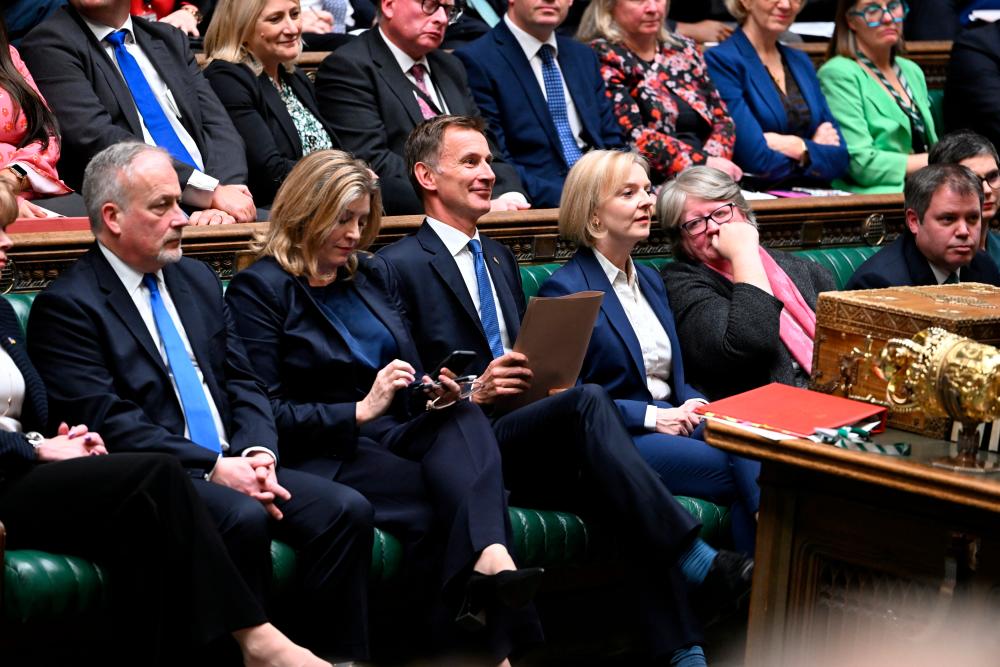The photo depicts a group of people seated in a tiered auditorium setup, akin to a courtroom or seminar hall, characterized by rows of seats that ascend gradually. In the foreground, on the right side, there is a wooden table containing various antique items including a brown box, a basket, and perhaps a red notebook.

In the first row, which is directly at ground level, there are eight individuals seated on what appears to be a long green leather bench. The gender distribution alternates between men and women. Most of the men are dressed in dark suits with white shirts and blue ties, and the women wear dark jackets over white shirts, with one woman notably sporting a pink scarf. One man with brown hair and a dark jacket is leaning forward, covering part of the face of a neighboring woman. Noteworthy expressions include a man in the front who is smiling broadly, almost on the verge of laughter, and a woman with highlighted shoulder-length hair who is leaning over, seemingly focused on her phone. Another woman in the front row has gray hair, while yet another has blonde hair.

In the second row, seven people can be distinctly seen from the waist up. The men are also clad in business suits similar to those in the first row. Among the women in this row, one wears a multicolored red, black, and white jacket, another sports a blue jacket with a black shirt underneath, and a third has a light green jacket. One woman mirrors the smile of the man directly in front of her, suggesting some amusement, but the rest of the group's expressions range from neutral to slightly amused.

Overall, the attire suggests a formal event, possibly an auction or seminar, given the professional clothing and the presence of the antique items on the table.